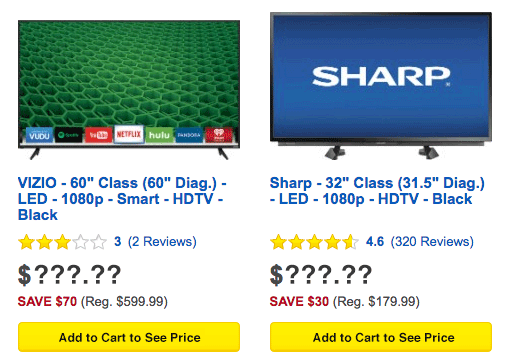This image displays two side-by-side advertisements for televisions available for online purchase. 

**Left Image**: The left section features a Vizio 60-inch Class LED Smart HDTV with a resolution of 1080p. The TV display showcases a green and dark green honeycomb pattern. Along the bottom, multiple streaming service logos are visible, including Hulu, Netflix, Vudu, and YouTube, among others. The product description below the TV reads: "Vizio 60-inch Class (60-inch diagonal) LED 1080p Smart HDTV - Black," all in blue text. The review section indicates the TV has received three out of five stars based on two reviews. The price is obscured with a dollar sign followed by five question marks. Below, a red text highlights a $70 saving, with the regular price listed as $599.99. A yellow box at the bottom with black text instructs users to "add to cart to see price."

**Right Image**: The right section showcases a Sharp TV with a black border. The TV screen is predominantly blue with the word "Sharp" written in white text. Specific details about this TV are not provided in the image description.

Overall, this side-by-side comparison appears to promote online sales for these two TV models.